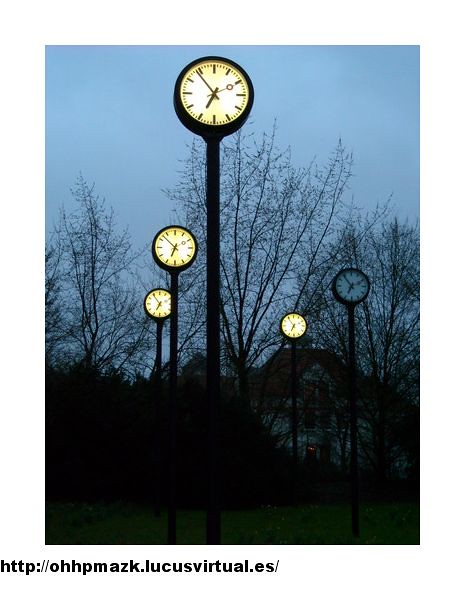The image showcases a color photograph taken at dawn or dusk, featuring five tall, old-fashioned analog clocks set against a backdrop of leafless winter trees, suggesting the winter season. Each clock is mounted on a slender black pole, and while four of the clocks are backlit with a soft yellowish-white glow, the clock on the far right lacks illumination. The simplified clock faces display the time—five minutes to seven—using only hour, minute, and second hands without numerical indicators. Below this scene, a partially visible website URL, http://ohhpmazk.lucusvirtual.es/, suggests a Spanish origin. In the lower right portion of the image, beyond the barren trees, sits a large mansion-like house, partially visible with a light-colored rooftop. The entire image, which is taller than it is wide, seamlessly merges into a white background.